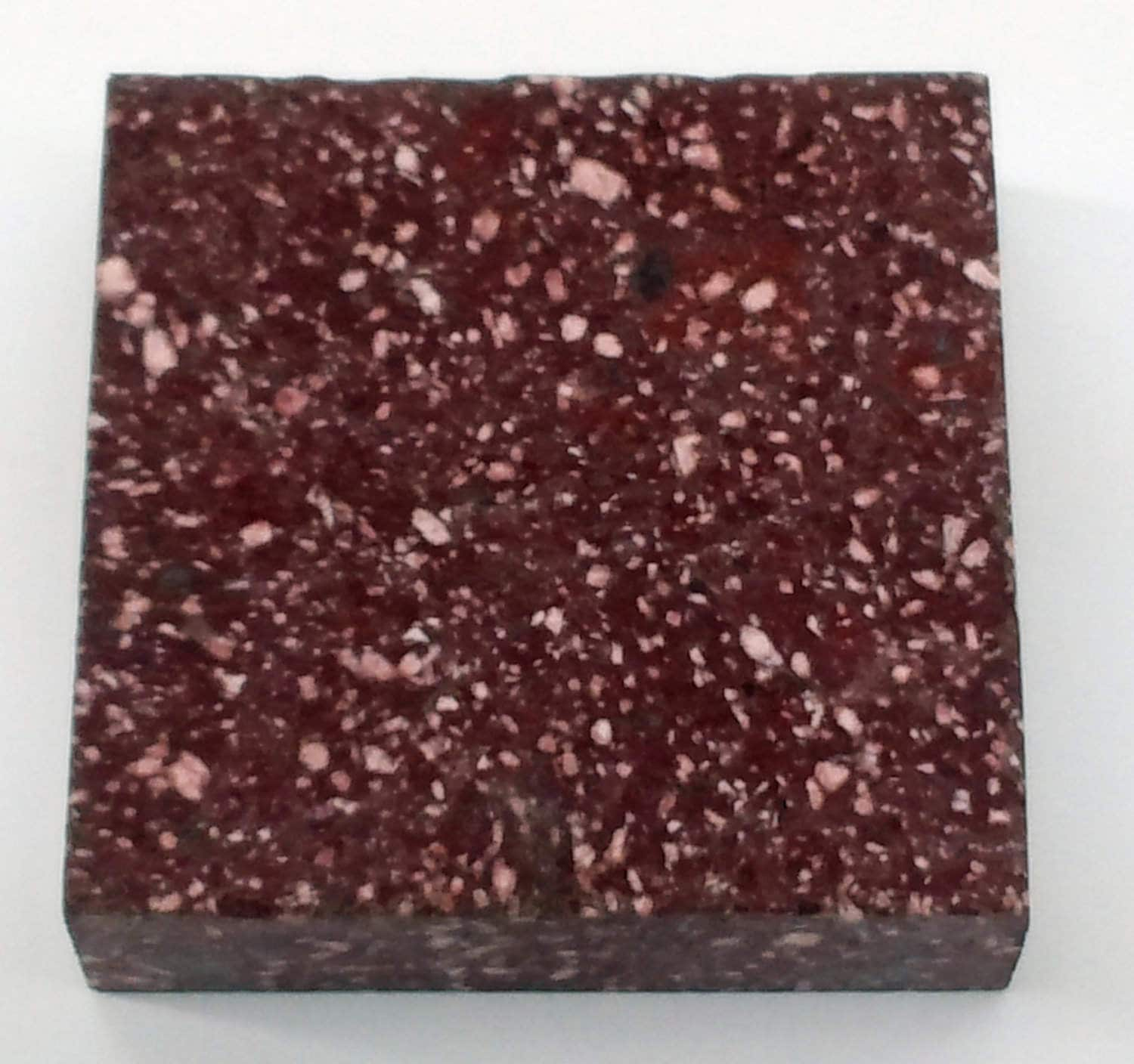The image depicts a detailed, zoomed-in view of a dark reddish-brown, 3D square block, covered in numerous white and black flecks of various sizes. The block has a rough, coarse texture, giving it an appearance that could be likened to a piece of rubber, granite, or even a type of food such as a brownie. The edges of the block are smooth and sharp, clearly defined against a grayish-white background with a slight shadow near the bottom, indicating the top-down perspective from which the photograph was taken. The object's dimensions and thickness are visible although no scale is provided, causing ambiguity about its actual size.